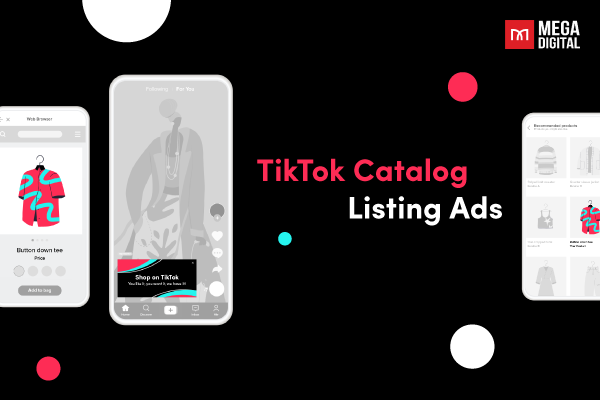Here is the cleaned-up and detailed descriptive caption for the image:

---

The image is a screenshot of an advertisement with a sleek black background, adorned with various circular patterns in different colors, including white, red, and light blue. Positioned at the top right corner, the word "MEGADIGITAL" is prominently displayed in block white letters. Adjacent to it on the left is MEGADIGITAL's logo, a red box featuring a white 'M'. 

The advertisement showcases three smartphone screenshots. The first screenshot features a red vacation-style shirt with light blue squiggly lines, hanging on a hanger. The second screenshot is larger and more central, depicting a stylish woman dressed in a gray coat, pants, crop top, and a necklace, with a highlighted rectangular bar at the bottom. The third screenshot displays various items in gray, similar to the grayscale aesthetic of the second image, with one item standing out — a shirt that mirrors the design from the first screenshot.

Centered within the advertisement, the words “TICSOC catalog” are presented in bold red text, accompanied by the phrase “listing ads” in white.